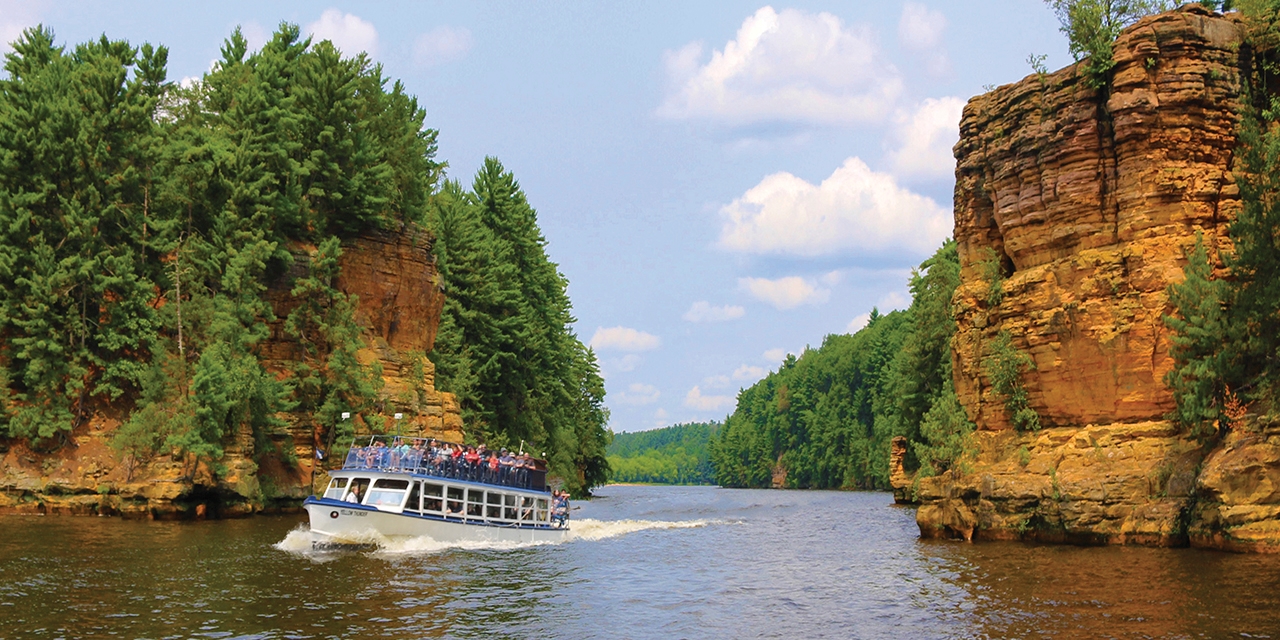In the image, a white and blue distinguished tour boat navigates through a vast waterway that exhibits a dark, almost brownish hue. The boat features numerous windows and a bustling top deck where many passengers are visible, enjoying the open air behind a safety railing. The vessel appears slightly tilted, with the rear more submerged than the front, creating a noticeable trail in the water. On either side of the waterway, towering cliffs rise dramatically, their red clay backgrounds adorned with lush green trees and vegetation. These imposing rock faces, several times the height of the boat, make the tour boat look small in comparison. In the background, a forest stretches endlessly, complementing the picturesque landscape. The scene is set under a broad daylight, with a clear blue sky interspersed with fluffy clouds, encapsulating the serenity and grandeur of nature.